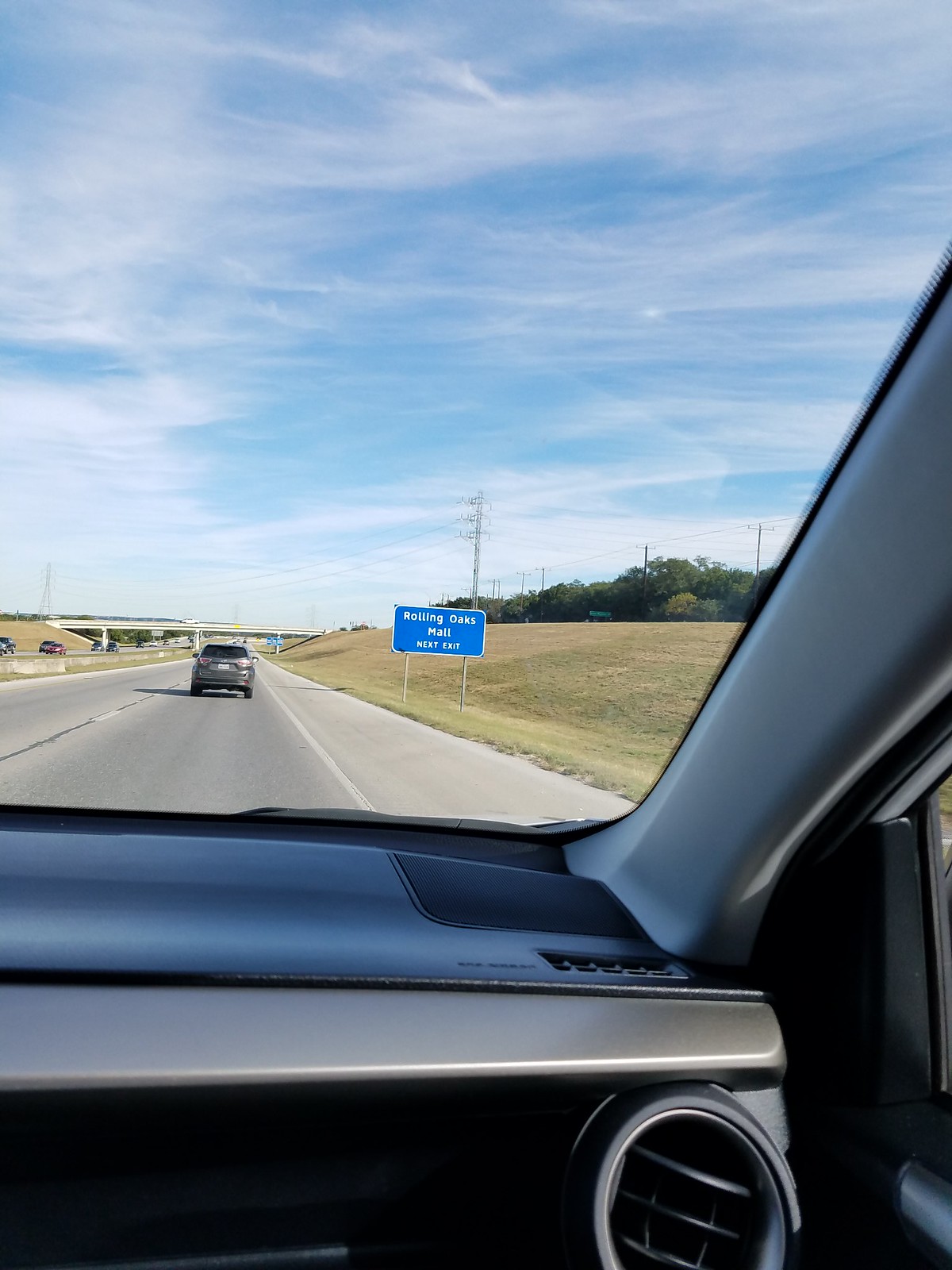This photograph, taken from the front passenger seat of a vehicle driving down an American freeway, captures a detailed and clean scene. The viewer looks through a pristine windshield onto a black-topped road, leading towards a blue sign which reads “Rolling Oaks Mall Next Exit.” Ahead, another road sign for restaurants or fuel stations can be seen, though its details are indiscernible from this distance. Right in front is a gray SUV, while on the right side of the frame, rolling hills with brown grass meet a few scattered trees and some electric wires supported by towers. An overpass looms further ahead. The sky above dominates the upper half of the image, showcasing a beautiful, powdery mix of blue and white clouds. Inside the vehicle, the interior's black dashboard, adorned with a silver accent piece and a circular, open air conditioner vent, is notably clean and shiny.